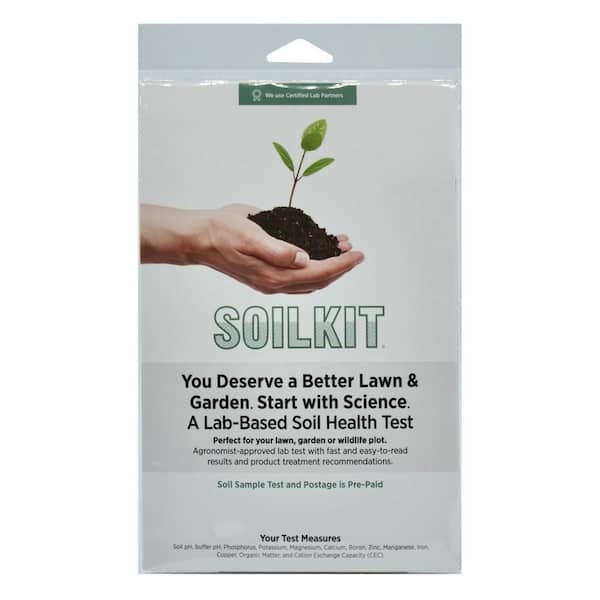The image showcases the front of a rectangular, light grayish-green package labeled "Soil Kit." Prominently featured in the middle is a photograph of two hands gently cupping a bundle of soil from which a small plant is sprouting. Below this image, bold black text reads, "You Deserve a Better Lawn and Garden. Start with Science. A Lab-Based Soil Health Test." Additional text provides further details, highlighting that the kit is "Perfect for Your Lawn, Garden, or Wildlife Plot" and is an "Agronomist Approved Lab Test with Fast and Easy-to-Read Results and Product Treatment Recommendations." The package also notes that the soil sample test includes prepaid postage and provides instructions on where to send the sample. The entire package appears sleek and has a designated tab for hanging.